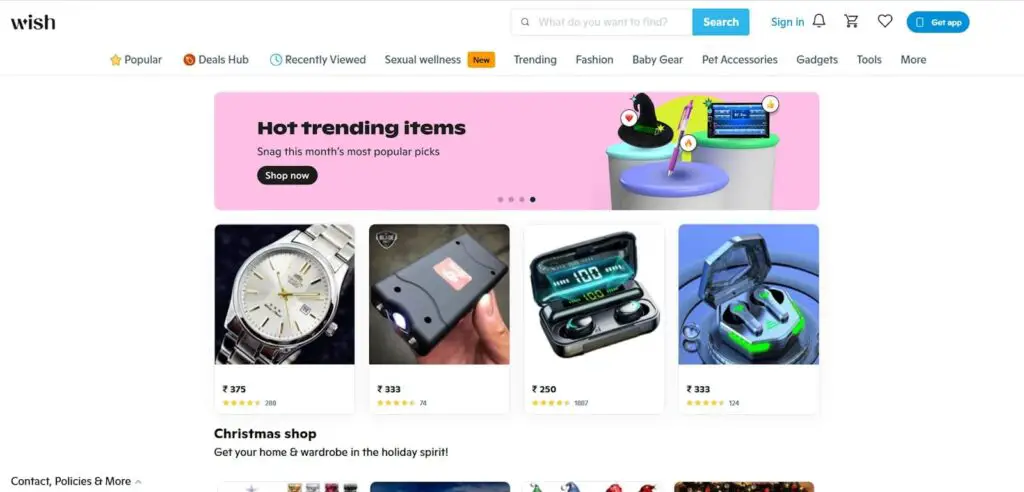This is a screenshot from the Wish.com website, showcasing various products available for purchase. The site's layout is predominantly white, creating a clean and minimalist aesthetic. In the top left corner, the "Wish" logo is prominently displayed in black. Towards the center-right of the page, there is a user-friendly search bar featuring a blue search button, designed to facilitate product searches.

Directly below the search bar, a navigation bar spans the width of the page, containing 11 distinct links for easy access to different sections of the website. Below the navigation bar, there is a pink rectangular section labeled "Hot Trending Items," drawing attention to popular products.

Further down the page, four product listings are displayed, each accompanied by a clear image. The first product is a stylish watch. The second listing features a taser, designed for personal safety. The third item is a pair of Bluetooth headphones, ideal for wireless audio convenience. The final featured product is another set of Bluetooth headphones, presumably differing in style or brand from the previous pair.